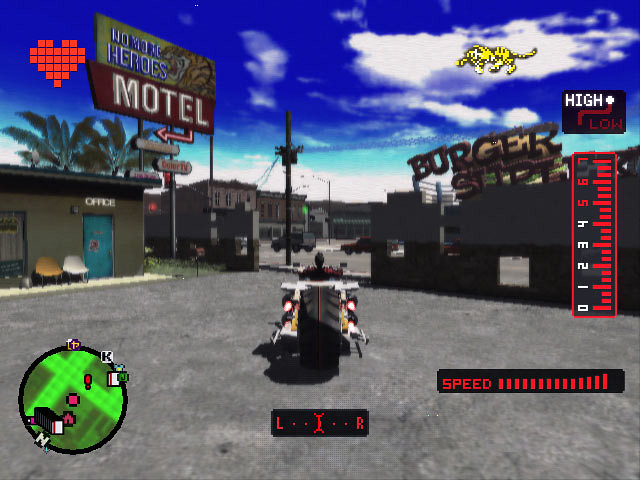The image depicts a screenshot from a video game, likely resembling GTA in style, possibly on a PS2 or PS3 platform. The scene is set in a parking lot adjacent to the "No More Heroes Motel," indicated by a large billboard in the top left corner of the screen, accompanied by a red pixelated heart suggesting the player's health. The central focus is a little avatar riding an oversized motorcycle with a disproportionately large back wheel. This futuristic motorcycle is equipped with various gadgets like wings and rockets. 

To the bottom left, there's a small green map, possibly a compass showing the player's location and direction. The right side of the screen features a digital display with indicators for speed, showing various gear levels from 0 to 7, where higher gears are marked in red, and the options for low and high speeds. Above this, a "Burger Something" sign is partially visible, hinting at a burger restaurant nearby, further detailed by a giant burger graphic. The background reveals blue skies with white clouds, buildings, power lines, and a wooden pole that connects these power lines, enhancing the scene's immersive and somewhat cartoony style. The overall visual is a blend of detailed game elements against a potentially realistic or well-rendered game environment, emphasizing the game's unique aesthetic and interactive features.